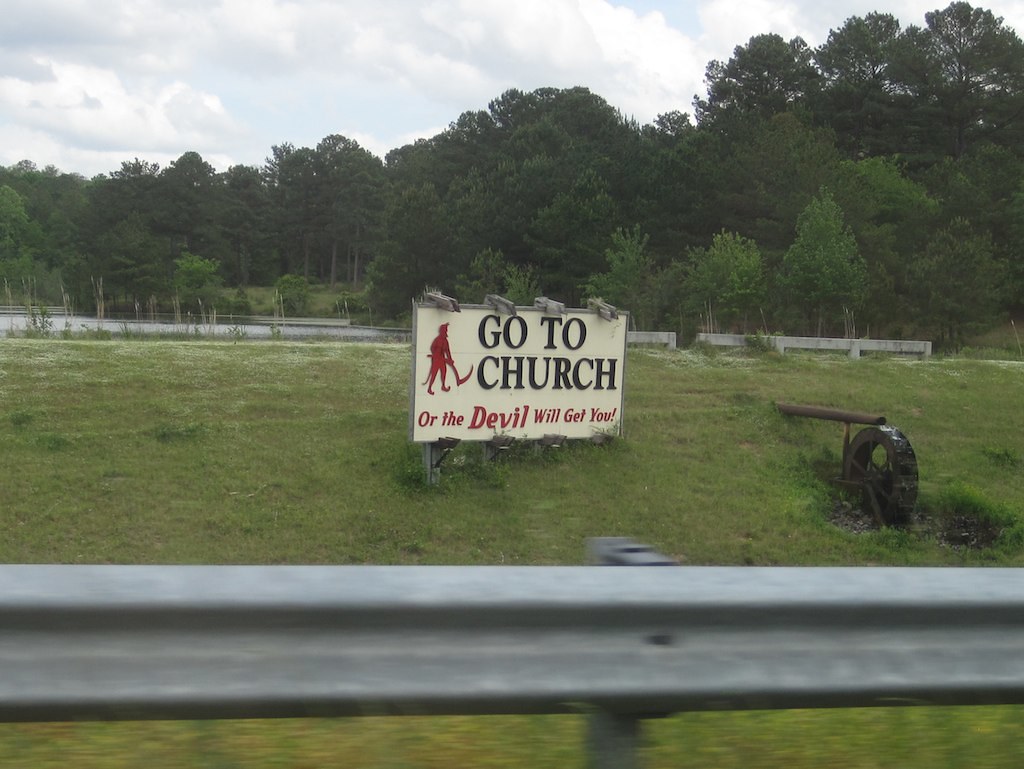The photograph appears to have been taken from a moving vehicle, evidenced by the slight blur and angle. The image prominently features a gray guardrail in the foreground, behind which lies a patch of green grass. Beyond the grass stands a rectangular, white billboard with striking black text that reads, "Go to Church." To the left of this text, there's a depiction of a red devil, accentuating the warning message. Below, in bold letters, the billboard continues with the phrase, "or the Devil will get you!" punctuated with an exclamation mark for emphasis. To the right of the billboard is an intriguing water fountain designed to resemble a wagon wheel, with a pipe directing water onto the wheel. In the background, a dense cluster of dark and light green trees completes the scene, providing a natural backdrop to this roadside message.